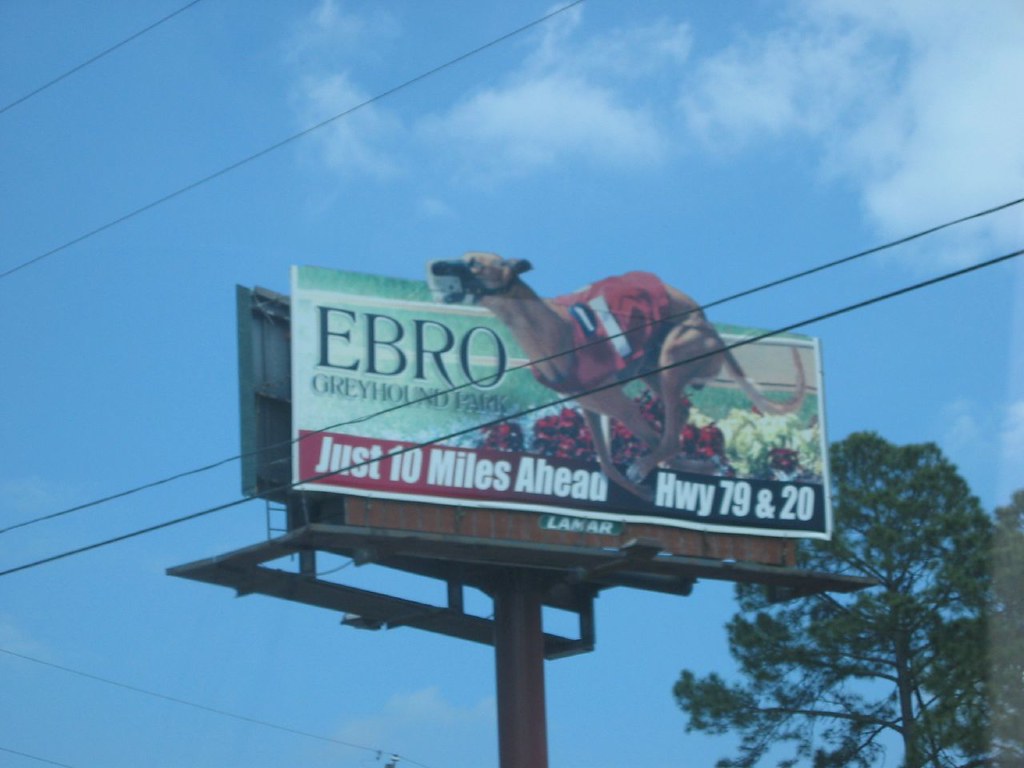The image captures a first-person perspective of an outdoor billboard, slightly offset to the left and angled upward, such that the ground and distant scenery are not visible. The sky dominates the background, mostly blue with some clouds creeping into the frame from the top right and top middle. Power lines traverse the scene, intersecting and overlapping the billboard. In the bottom right corner, a tree peeks into the frame, rising behind the billboard.

The billboard itself is supported by a singular cylindrical brown pole. The main graphic on the billboard features a greyhound dog, distinctly drawn and adorned with a jacket or saddle. The dog also appears to be equipped with a muzzle. To the left of the greyhound image, the word "Ebro," spelled E-B-R-O, is prominently displayed. Below this, the word "greyhound" labels the dog.

At the bottom of the billboard, a red banner displays the message "just 10 miles ahead, HWY 79 and 20," directing travelers to a nearby location. The small rectangular writing attached to the billboard frame reveals the brand, "Lamar," spelled L-A-M-A-R.